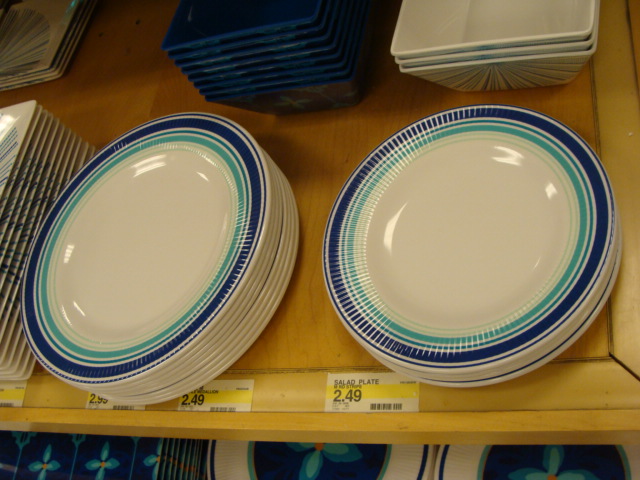The image depicts a display of various plates and bowls arranged on a light-colored wooden table or shelf, likely at a Target store as indicated by the style of the price tags. In the lower part of the image, there are two stacks of salad plates positioned on the right and left sides. The plates are predominantly white or off-white with a decorative pattern consisting of multiple concentric rings in shades of navy blue, teal, and light green. The innermost portion of the plates remains plain white. 

The salad plates on the right side of the display are priced at $2.49 each and feature four or five plates in a stack. On the left, there are approximately eight slightly larger plates, potentially dinner plates, bearing the same pattern; their price tag reads $2.99. Above these stacks, towards the top of the image, there are several square-shaped bowls. On the right side, there are three white and blue bowls with a starburst pattern. On the left side, a stack of approximately nine navy-blue bowls can be seen. Additionally, there are some flat, square plates on the far left, matching the color scheme but displaying a slightly different pattern from the concentric-ringed plates.